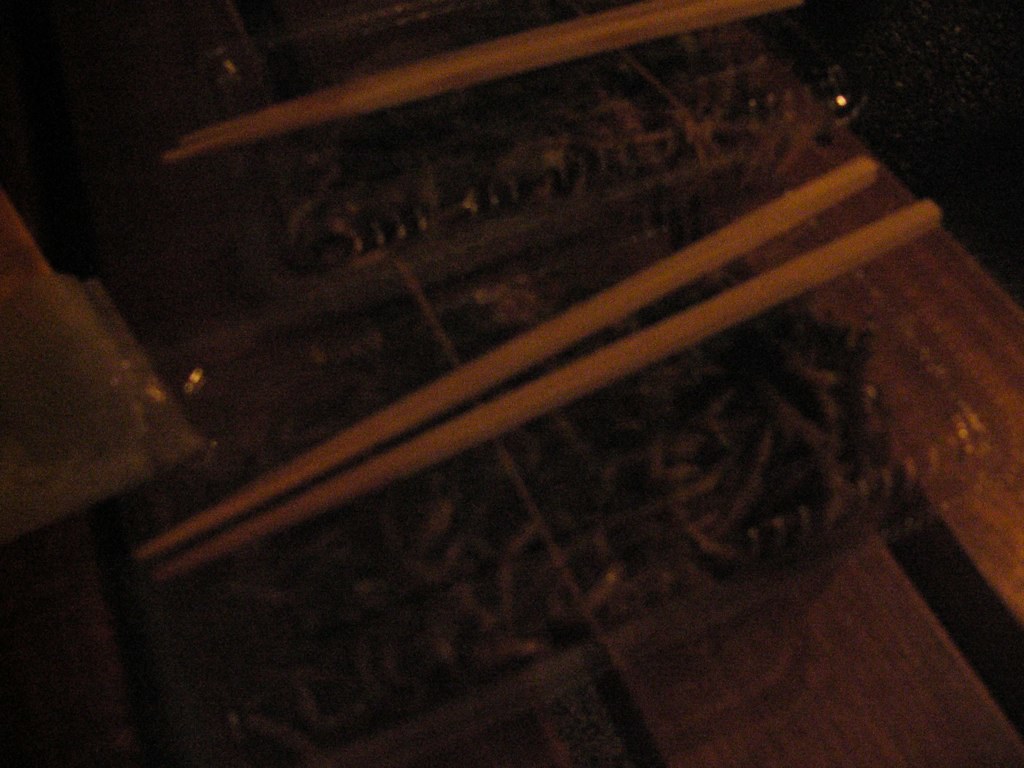This digital photo showcases a dark and somewhat blurry scene centered around a wooden picnic table or chair, characterized by its extremely dark brown hue. The right side of the photograph fades into nearly complete blackness, adding to the overall dim ambiance. Positioned centrally and towards the upper portion of the image are two plastic containers arranged one in front of the other. Each container is closed and has a pair of light brown, wooden chopsticks resting on top. The containers appear to hold a dish resembling long, skinny noodles in a brown sauce, likely an Asian noodle dish. The container toward the back features black text, though it's illegible. Additionally, both containers seem to have a rubber band wrapped around their middles, securing them.